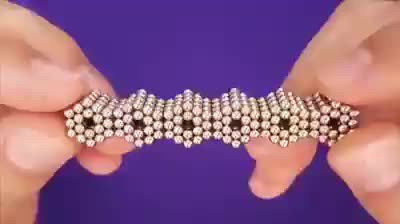The image features a close-up of the fingers of two hands, each gently holding a metallic object made of smaller segments. The object, appearing like a piece of jewelry or intricate metallic construction, consists of six hexagonal segments, each formed by tiny metal beads or magnets. These hexagons are aligned next to each other, and each has a small hole in its center. The background is predominantly blue, adding contrast to the metallic shine of the object. The overall composition highlights the delicate nature of the hands and the intricacy of the metal object they are holding.